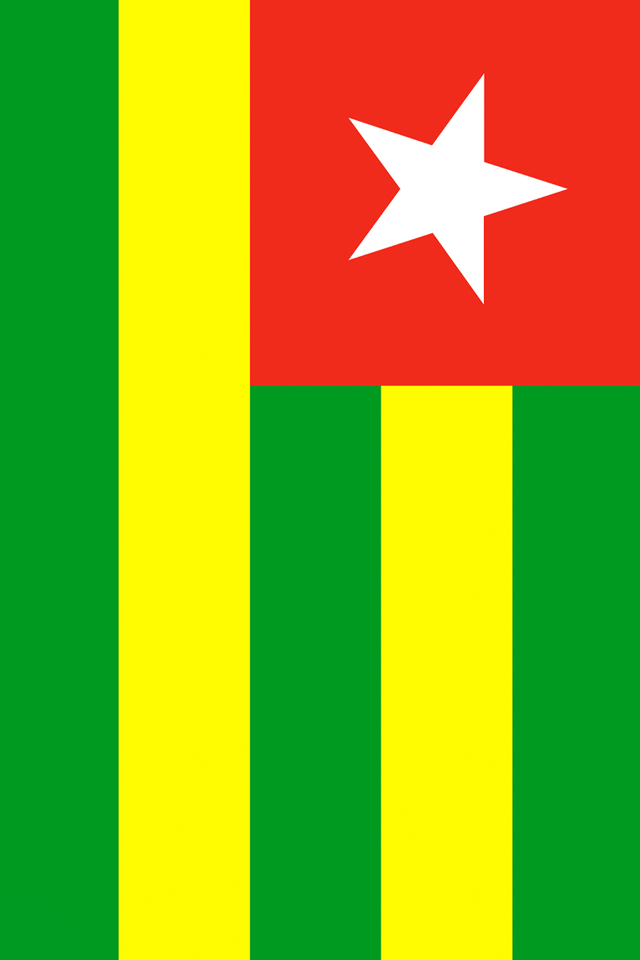This is a vertical, digitally generated image of a flag featuring four primary colors: red, white, green, and yellow. The upper left portion of the flag has a prominent red square with a white star at its center. Surrounding the red square, the flag is adorned with five stripes in total: three green and two yellow. The arrangement of the stripes from top to bottom is green, yellow, green, yellow, green. The top three stripes cover roughly two-thirds of the flag's width, whereas the bottom two stripes extend across the full width. The flag's design includes basic geometrical shapes, creating an orderly and symmetrical appearance. There is no text or other symbols within the flag, and it is displayed on a simple white background.